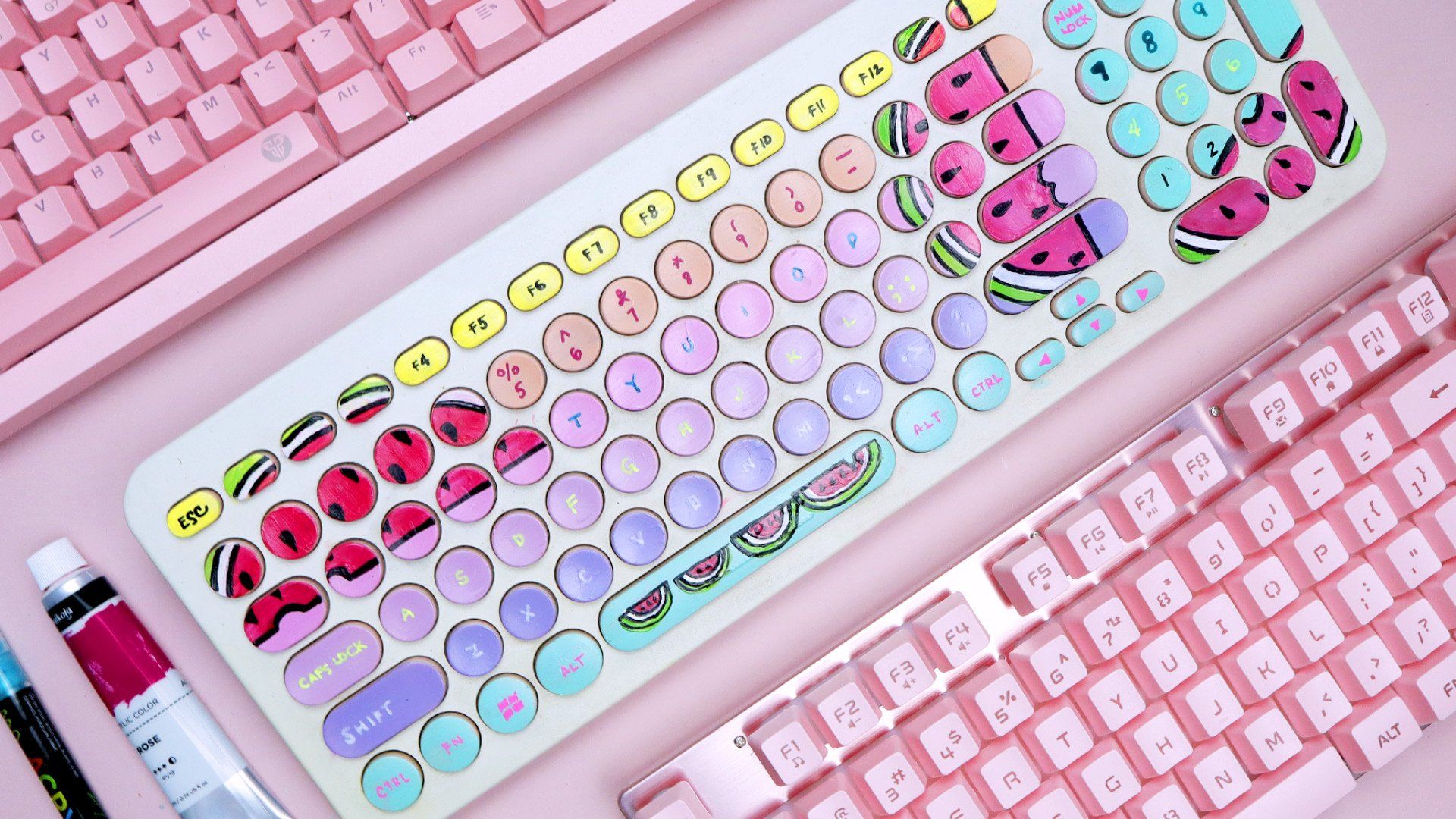In this rectangular photograph, measuring approximately 6 inches wide by 3 inches high, we see three computer keyboards arranged diagonally from the upper left to the lower right. The dominant color of the image is pink. The keyboards create a cascade down the frame, with the topmost and bottommost keyboards partially cropped from view. 

The keyboard in the upper left corner is a bright pink color. We can see a section including the space bar, Alt key, and some F keys before it trails off the screen. The central keyboard is a white one, adorned with a colorful array of keys painted in pastel hues: pink, lavender, violet, turquoise, light blue, and peach. Some keys are illustrated to resemble watermelon slices, adding a whimsical touch. The keys also have a gradient effect, fading from darker to lighter shades of purple and pink, with a few yellow buttons scattered throughout.

The bottom right keyboard is light pink, with its sides extending beyond the photograph's edges, similar to the top keyboard. To the left of the central white keyboard, there appears to be a tube of red paint and potentially a blue or black marker, suggesting that the colorful keys might have been custom-painted.